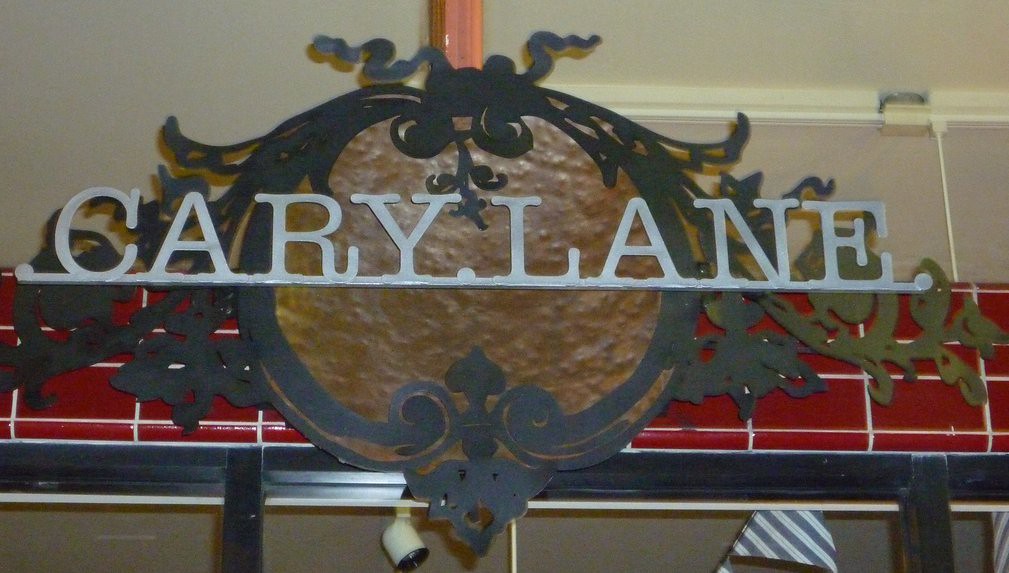The image showcases a detailed and ornate decorative piece mounted on a wall. The background features a mix of white and red tiles, with a section of pink tiles adding contrast. Below the tiles, there's a black windowsill border that frames a window pane. The focal point of the image is a unique, roundish knick-knack that bears an intricately designed leaf shape at the bottom, with black ornate lines and borders. This decorative piece, which evokes a whimsical flair reminiscent of Cinderella's pumpkin or an owl's face, is predominantly brown with a golden element at the back and additional leaf-like details on the right side. Across the center of the brown piece, the name "Carrie Lane" is inscribed in gray, bluish-whitish text, and it is underlined. Underneath this decoration, a black metal horizontal pole with vertical lines adds a touch of industrial charm.